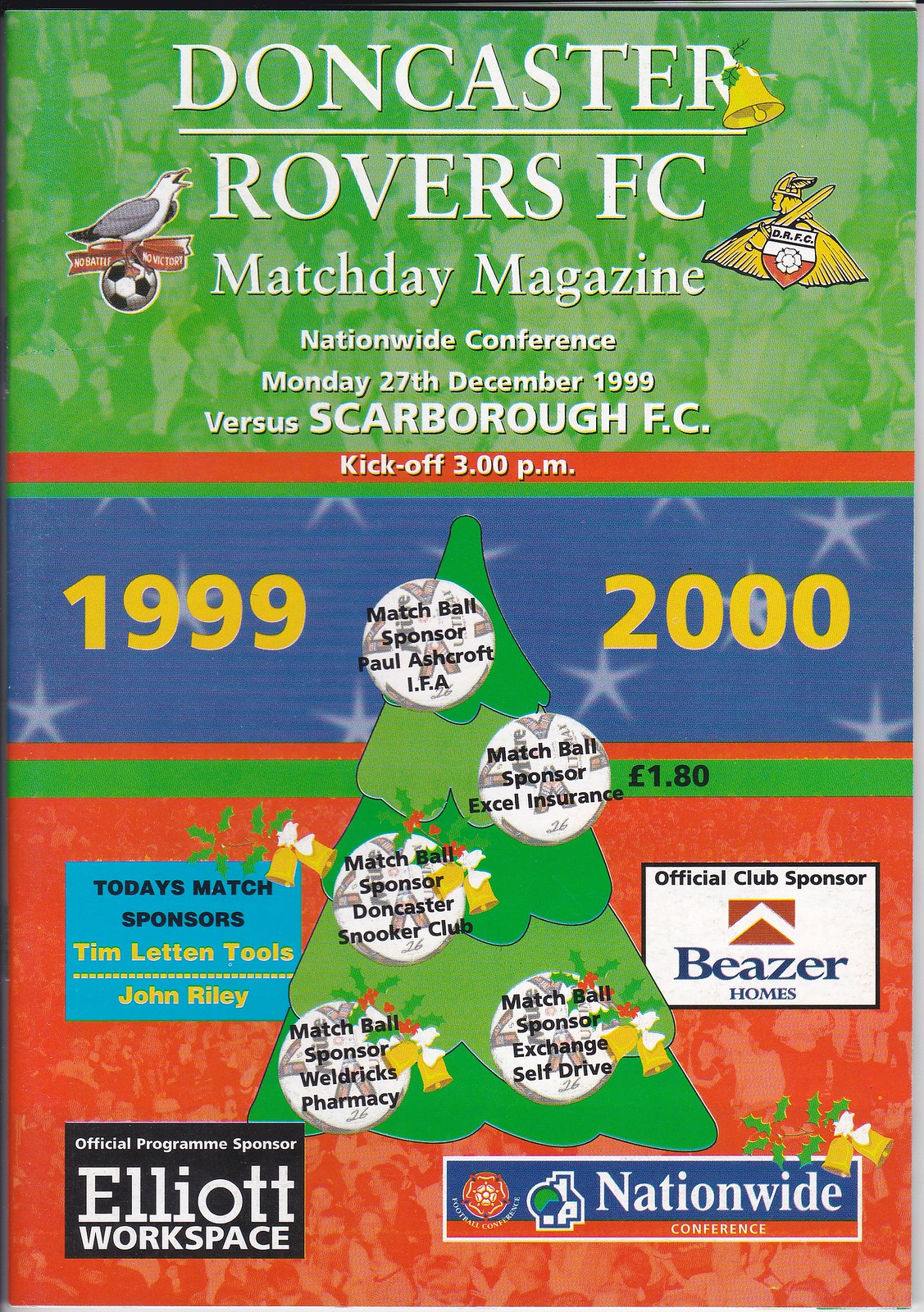The cover of the Doncaster Rovers FC Match Day Magazine for the Nationwide Conference match versus Scarborough FC on Monday, December 27th, 1999, features a colorful and festive design. The background is divided into three sections: light green at the top, blue in the middle, and red at the bottom. At the top, in the green section, the text reads "Doncaster Rovers FC, Match Day Magazine." Accompanying this text are a bird standing on a soccer ball to the left and images of a bell and a Viking with a shield to the right. 

The middle, blue section prominently displays "1999-2000" and features a large clipart-style Christmas tree decorated with soccer balls, extending into the red bottom section. Surrounding the base of the tree, there are various advertisements for sponsors such as Beezer Homes (official club sponsor), Nationwide Conference, Elliott Workplace, and others like XL Insurance and Weldrix Pharmacy. 

The cover also lists important details about the match, including the date and the teams playing, noting a kickoff time at 3 p.m., making it clear that this is a special Christmas-themed edition. The magazine's price is shown as $1.80. This vibrant and detailed cover merges holiday spirit with essential match and sponsor information, set against a festive and colorful backdrop.